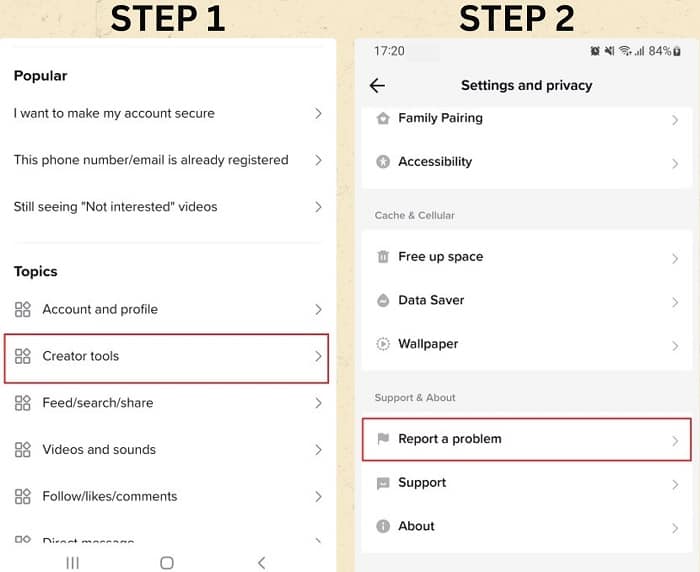This image features a detailed guide for securing an account, set against a pink background. The guide is presented across two mobile phone screens labeled as "Step 1" on the left device and "Step 2" on the right device.

On the left screen under "Step 1," there is a white background header stating "Popular," followed by a series of options all marked with right arrows:
- "I want to make my account secure"
- "The phone number/email is already registered"
- "Still Seeing Not Interested Videos"
- "Topics"
- "Account and Profile"

Highlighted within a red and blue box is "Creator Tools," followed by other options:
- "Feed"
- "Search"
- "Share"
- "Videos and Sounds"
- "Follows, Likes, and Comments"

On the right screen under "Step 2," the following elements are detailed:
- A light blue box displaying the number "1720" and a left arrow button labeled "Settings and Privacy"
- Below is a white box with options "Family Pairing" and "Accessibility," both marked with right arrows

Following these, the next set of options includes:
- "Cash and Cellular"
- "Free Up Space," "Data Saver," and "Wallpaper," each accompanied by right arrows
- "Support and About" with a right arrow, and another section boxed in red and blue lines labeled "Report a Problem" with a right arrow

At the bottom, "Support and About" options appear again, each marked with right arrows.

This thorough layout aids users in navigating through various settings and features relevant to account security and other functionalities.